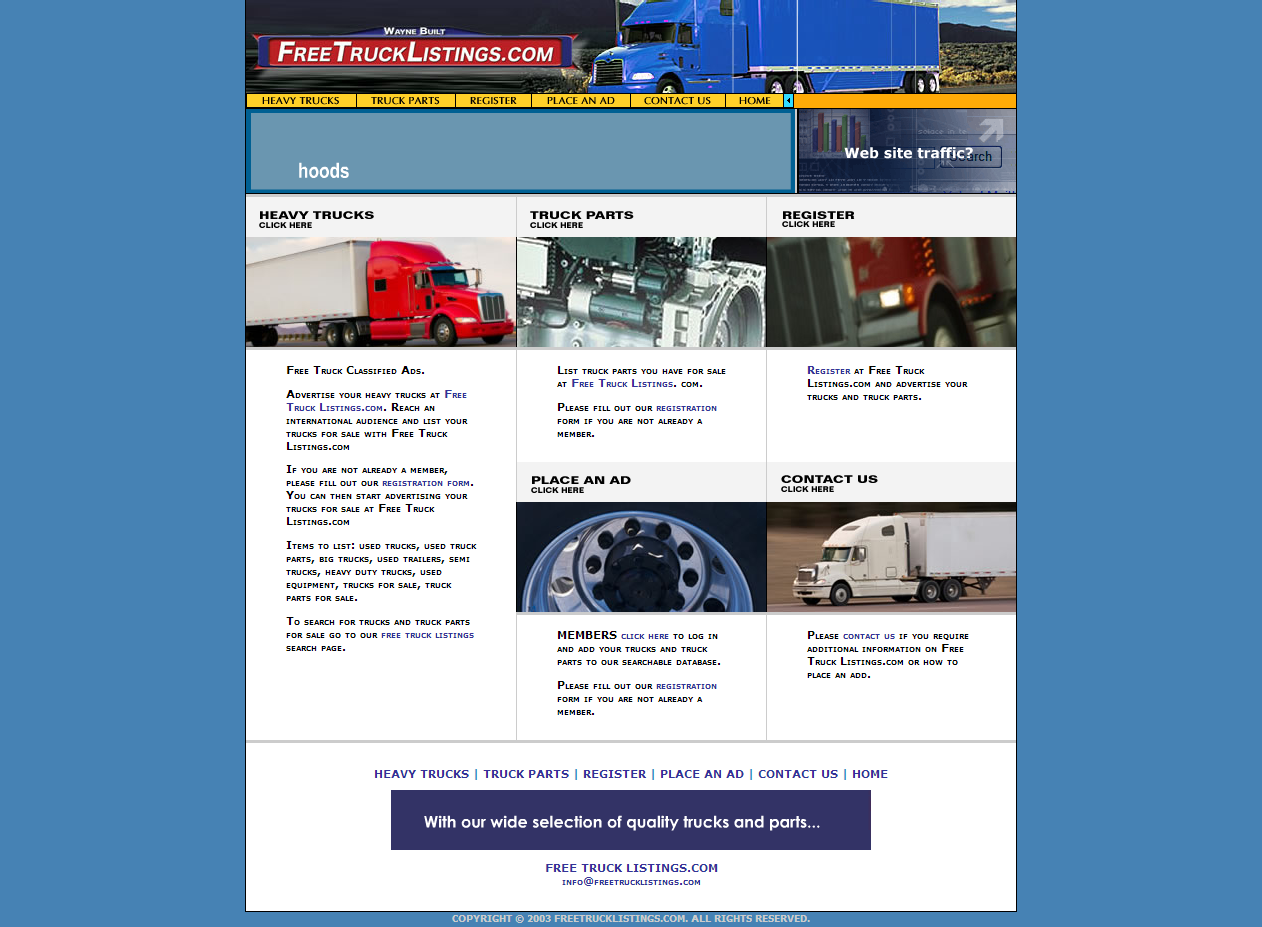Here is a detailed and cleaned-up caption for the image:

---

The image features a medium-tone blue background. At the top, there is a horizontal red rectangle with the text "FREE TRUCK LISTINGS.COM" in all capital letters, formatted in a white font with the first letter of each word bolded. To the right of the text, there's a picture of a Royal blue truck facing toward the left.

Below this red rectangle, there is a menu bar with a yellow background that lists several items in all capital, dark-colored font: "HEAVY TRUCKS," "TRUCKS AND PARTS," "REGISTER," "PLACE AN AD," "CONTACT US," and "HOME."

Under the menu bar, there is a lighter blue horizontal rectangle running three quarters of the way across the page to the right edge. Within this light blue area, there is white text asking, "WEBSITE TRAFFIC?" accompanied by an arrow pointing to the upper right corner.

On the left side of the lighter blue rectangle, the word "HOODS" is written in white font slightly in from the left edge. Below this section, the background of the page turns white.

The white portion of the page includes several clickable sections:
- **Heavy Trucks**: Features an image of a large red and gray truck facing towards the right edge, with the text "CLICK HERE" in small black font underneath.
- **Truck Parts**: Displays an image of various truck parts with the text "CLICK HERE" also in small black font.
- **Register**: This section has the text "CLICK HERE" and is accompanied by an indistinct image that appears to include some machinery.
- **Place an Ad**: Another section with the same small "CLICK HERE" text and again, a somewhat unclear image of machinery.
- **Contact Us**: Shows a white truck driving towards the left edge, with "CLICK HERE" beneath it.

At the bottom of the page, there is a horizontal purple rectangle with white text stating "WITH OUR WIDE SELECTION OF QUALITY TRUCKS AND PARTS..." Directly above this text, in the same purple writing, are the menu items listed again: "HEAVY TRUCKS | TRUCK PARTS | REGISTER | PLACE AN AD | CONTACT US | HOME." Below this line, the text "FREE TRUCK LISTINGS.COM" appears once more in the same purple font.

---